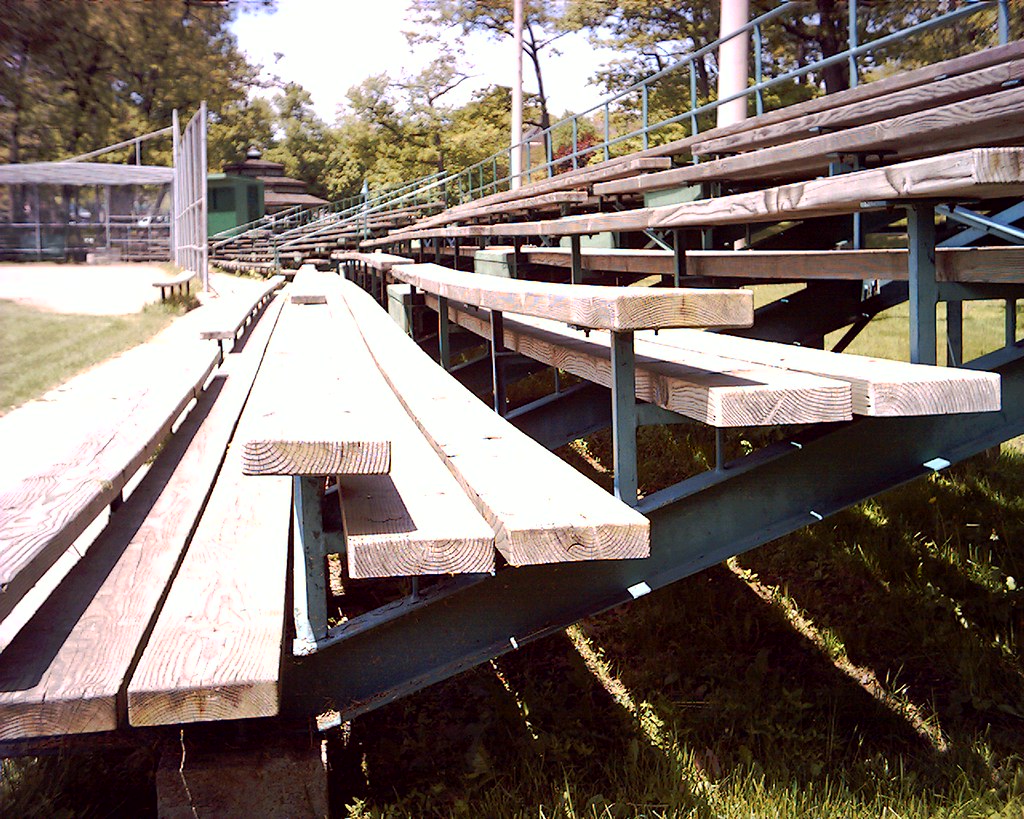The image depicts an empty set of wooden bleachers with a metal frame, located at a local baseball field surrounded by tall, leafy trees, possibly indicating the fall season with some leaves changing color. The photo is taken from the side, focusing on the bottom sections of the bleachers. A railing runs along the top of the stands and down one side, while the other side lacks a railing, providing easier access. In the far left corner, part of the baseball diamond is visible, including the home plate area and a bench for the players next to a high fence designed to protect the catcher from stray balls. Beyond the fence stands a green building with a gray roof, featuring a descending series of three roof sections, likely serving as restrooms. The setting is bright and clear, taken during the daytime under plenty of natural light, and there's a noticeable contrast between the light brown of the wooden seats and the green and metal framework of the bleachers. Further details include some faded light green grass and patches of dirt around the home plate area, enhancing the rustic and slightly worn appearance of the field.